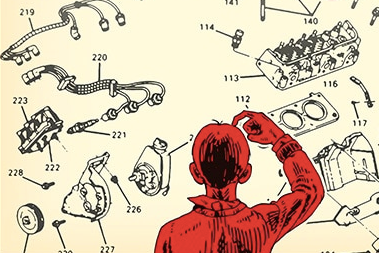The image appears to be an artistic drawing of a boy positioned slightly to the right of center. The boy is facing away from the viewer, showcasing the back of his head and upper body, which are rendered in a striking red color. The boy's figure is truncated just below the chest, revealing his right arm raised, as if he's scratching the top of his head in a contemplative manner. Surrounding the boy and dominating the rest of the yellow background are various car parts, each meticulously placed and labeled with lines and numbers. The parts seem to float in a sparse yet methodical arrangement, lending the whole composition a technical blueprint-like quality.